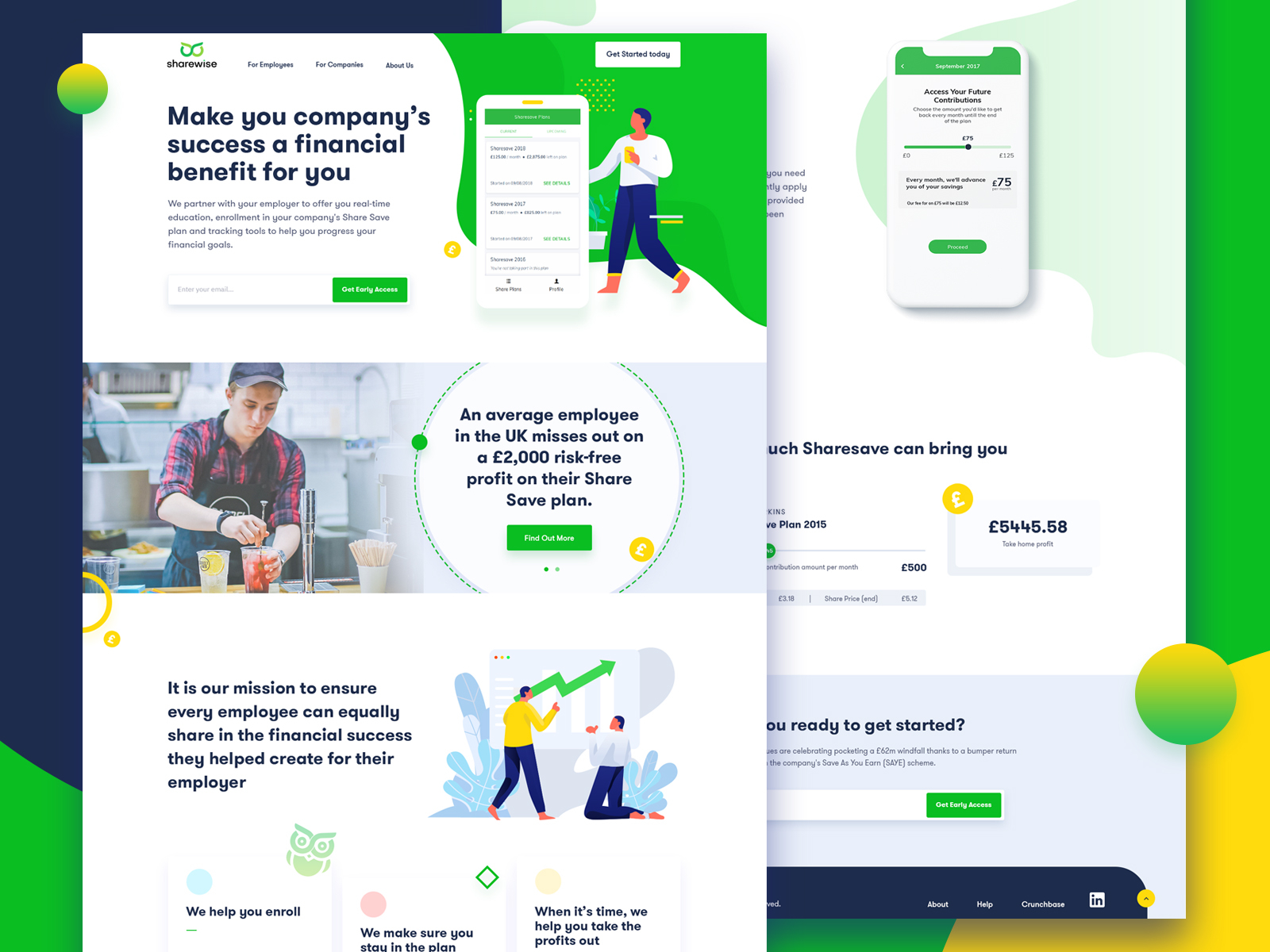This image resembles a corporate advertisement designed to inform employees about financial benefits. It features a dark blue half-square on the left that transitions into a white section, and then into a green square. On the left, there's a green and yellow circle with small text that’s hard to read. The text "Shorewise" is written beneath the green owl eyes graphic, accompanied by very small font.

To the right, a white square is filled with small text. Adjacent to it on the left, larger black text reads, "Maker Company, success of financial benefit for you," followed by tiny black text beneath, and a gray square further below. The area contains scattered green squares with white text.

Central to this section is an image of a smartphone with a green square at the top, portraying three white boxes filled with gray and green text. Below, a person in a white sweater, blue pants, and brown boots is pictured against a green background with white at their feet.

In another segment, an image shows a white male mixing a drink in a kitchen, wearing a blue cap, rolled-up sleeves, and overalls. A green dotted circle is on the right highlighting text that reads, "An average employee in the UK misses out on a 2,000-pound risk-free profit on their share save plan," enclosed in a green square with white lettering and an orange-circled pound symbol. The background is light blue, with the kitchen appearing grayish.

Below this, black text on a white box declares, "It is our mission to ensure every employee can equally share in the financial success they help create for their employer." To the right, a cartoon shows one person pointing at a flowchart, donned in an orange top and blue pants. Another individual in blue pants and a white top kneels, inspecting a pie chart with a green upward arrow against a gray background.

On the bottom left, there's a green image of an owl next to a blue circle, with a black text declaring, "We help you enroll," separated by a gray line from an orange circle and a tilted green square. Below the pink circle, the text, "We make sure you stay in the plan," is followed by another gray line separator and a beige circle with the text, "when it's time, we help you take the profits out." Yet another gray line separates this from a white phone-shaped box with a green square at the top, black and green text underneath detailing share save benefits potentially worth £5,445.58, with the pound symbol in an orange circle. A partially visible line indicates £500 to the left.

The bottom of the image features a blue background with the text, "Ready to get started?" in gray. There’s a white box beside a green box with white lettering, and a blue, almost square box at the bottom, possibly containing Indeed’s white logo. Overlaid text and symbols include a yellow circle outlined in green at the top, a yellow and greenish circle to the right, and an orange half-circle converged with green towards the center.